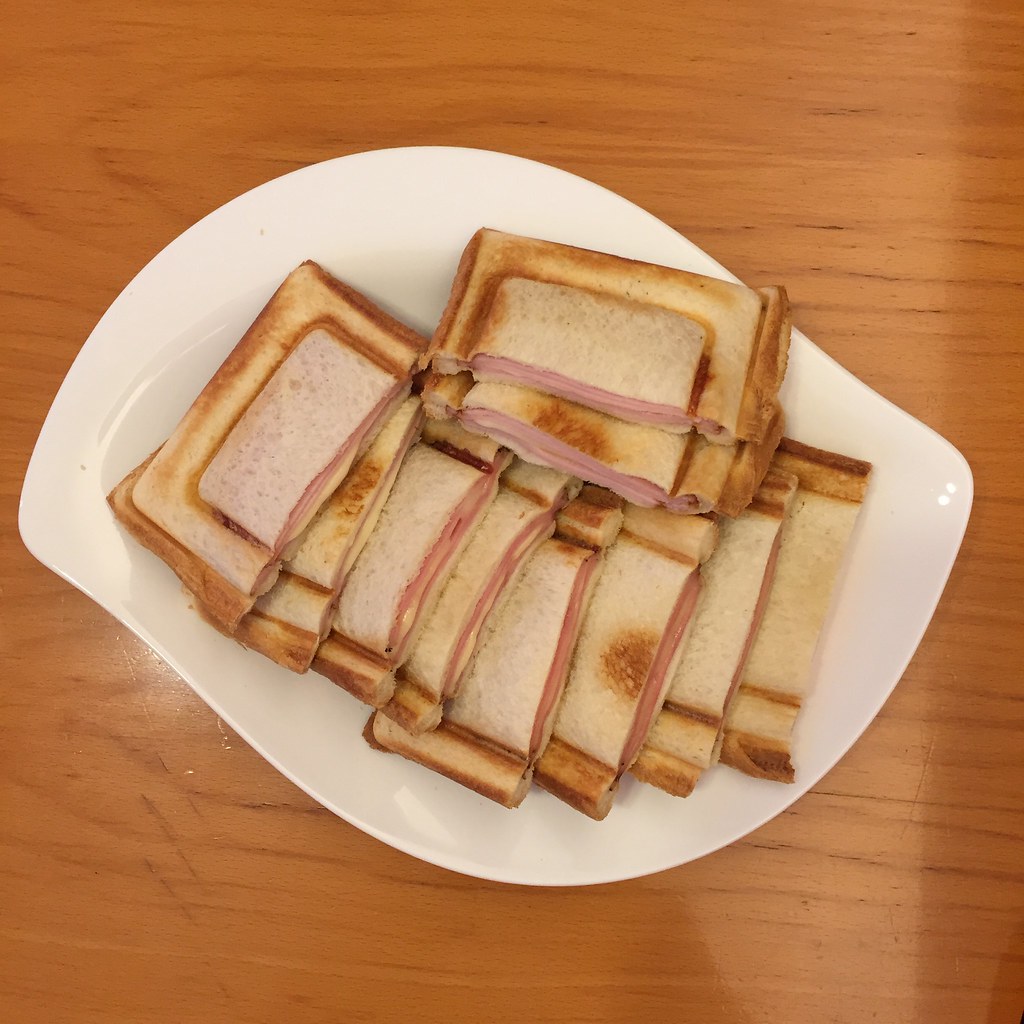The image showcases a distinctive, white, oblong-shaped platter with teardrop ends, resembling a stretched circle, set on a medium red-brown wood surface with visible grain details. The platter features a series of overlapping sandwiches, each cut in half and aligned uniformly. The sandwiches appear lightly toasted with grill scoring and crimped edges, suggesting a sealed, pocket-like structure. They contain a pinkish filling, likely deli ham, adding a touch of warmth to the lightly toasted bread, which may be either a light wheat or white bread. The absence of text or signatures keeps the focus on the culinary presentation.